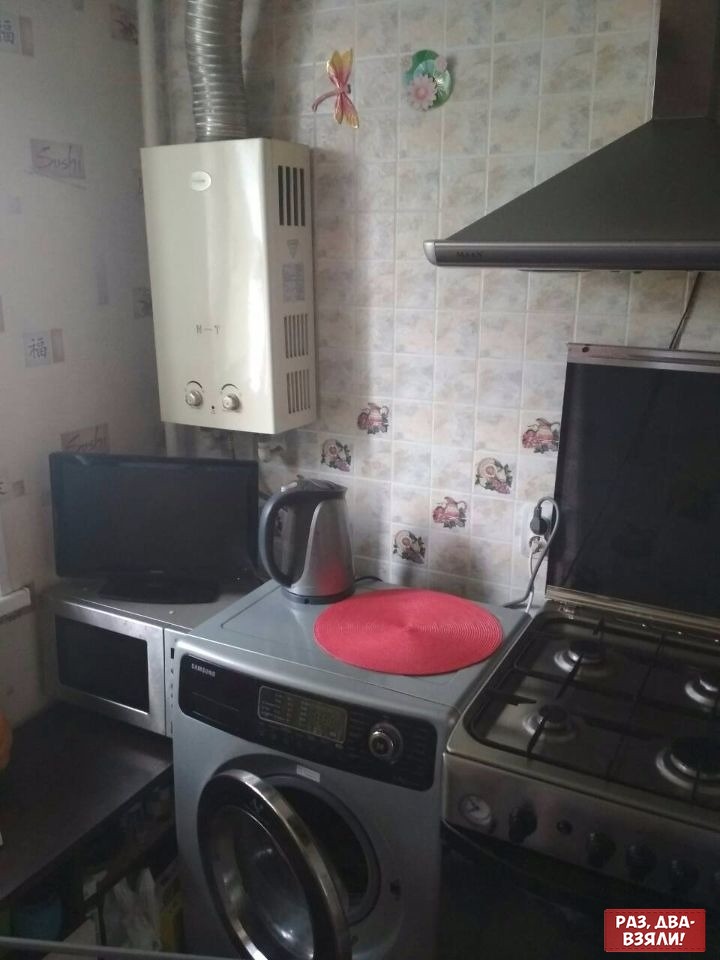The image depicts a cluttered kitchen with various appliances and decorations packed into a small space. The kitchen features old-fashioned linoleum tile and pale-colored floral wallpaper forming the backdrop, adding a quaint touch. Prominently on one wall, Chinese characters spell out "sushi," accompanied by a butterfly and a small decorative plate, contributing to an eclectic ambiance. In one corner of the kitchen, there's what looks to be an air conditioning unit.

At the heart of this compact kitchen, a silver microwave sits on a small bench or table with a black TV or computer monitor perched on top. To the left of the microwave, there's a gray, front-loading washing machine with its door open. A red mat and a tea kettle are placed on top of the washing machine, highlighting the multi-functional and densely packed nature of the space. The stove, black with four burners and an oven vent fan above it, is nestled closely beside the washing machine. An electrical outlet nearby is occupied with plugged-in devices, indicative of the space's busy utilization. In the bottom right-hand corner, a red rectangle with the inscription "PA3 ABA B3RAN!" is visible, adding a pop of color and curiosity to the scene.